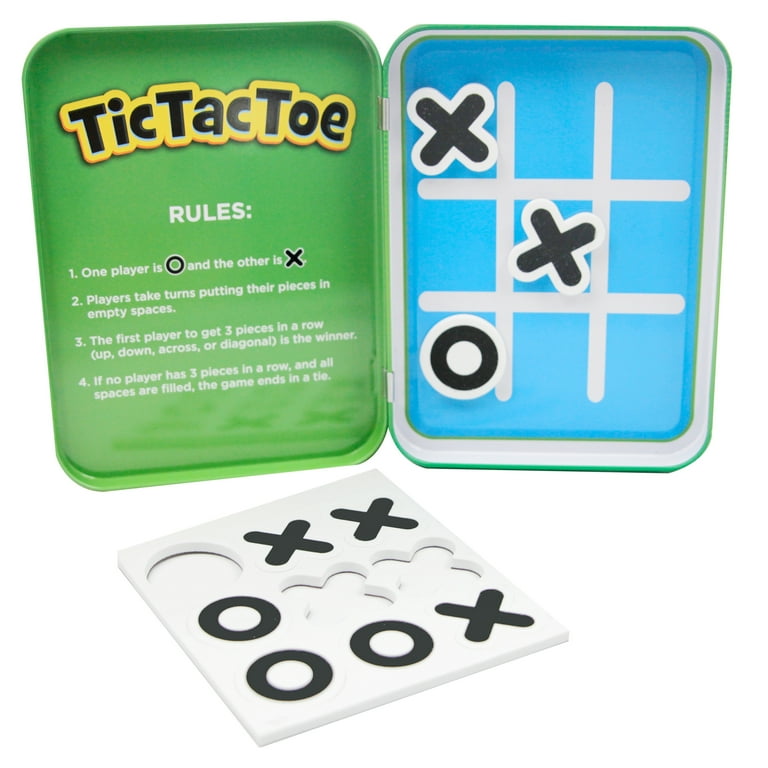The image depicts a vertically oriented scene against a white backdrop, showcasing a tic-tac-toe game with three distinct elements. At the top left, there is a green tin container with "Tic-Tac-Toe" written in bold orange letters, followed by the game rules in white text: 1. One player is O and the other is X. 2. Players take turns placing their pieces in empty spaces. 3. The first to align three pieces in a row—vertically, horizontally, or diagonally—wins. 4. If no player achieves this and all spaces are filled, the game results in a tie. On the top right, a blue and white box functions as the storage for the X and O pieces, which are made of plastic. Below these containers, the tic-tac-toe board itself is displayed: it has a blue background with white gridlines. Most of the pieces are already in place, with a black X in the top left, a black X in the center, and a white-bordered black O in the bottom left. In front of the board, additional pieces—two black X’s and one white-bordered black O—are laid out, ready to be placed in the remaining spaces.